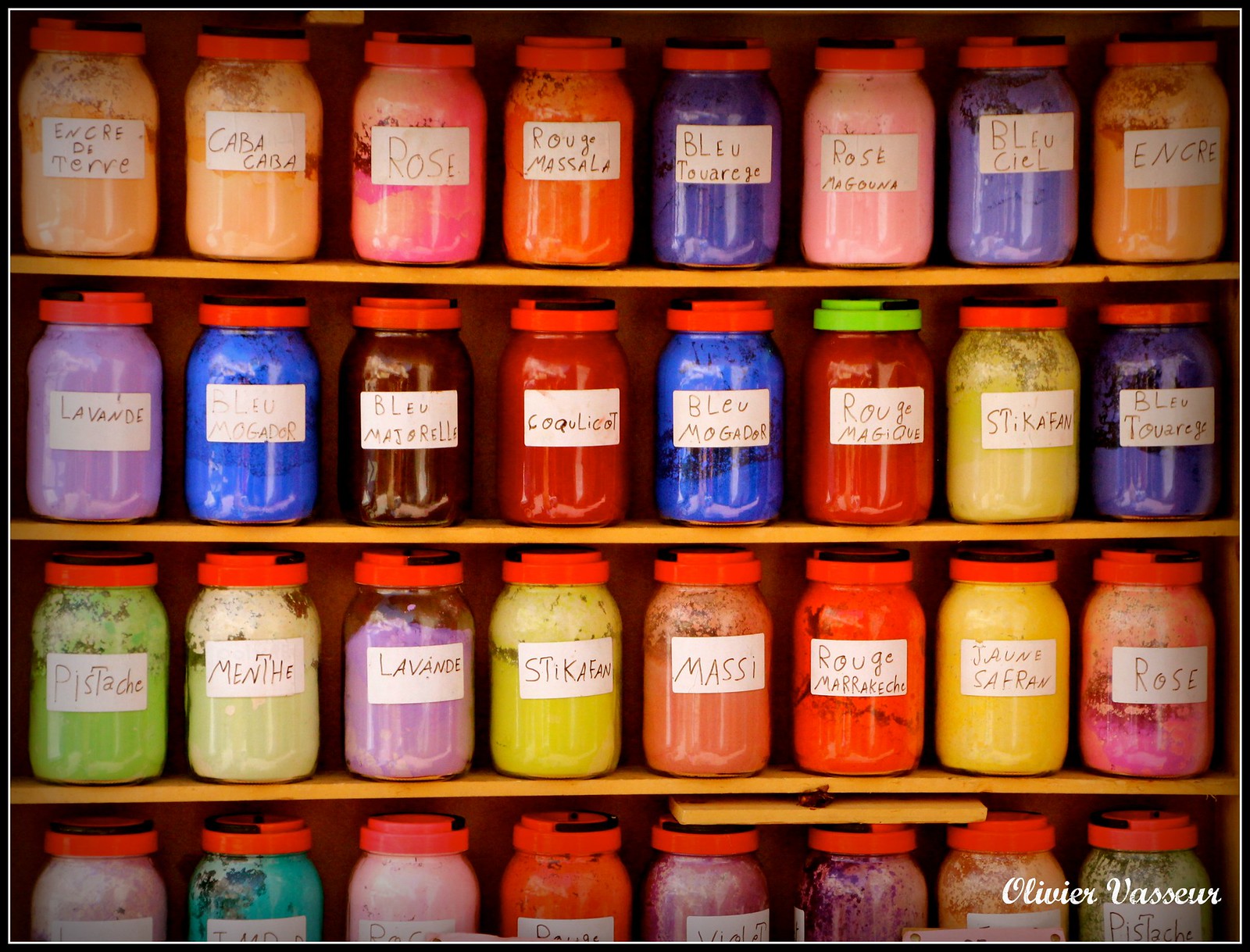The image features four light orange-colored shelves, each lined with a total of 32 vividly colored mason jars. These jars are filled with various brightly hued powders—ranging from peach, deep orange, hot pink rose, light pink, lavender, deep purple, indigo blue, yellow, green, turquoise, and other shades of purple. Each jar is adorned with a handwritten white rectangular label indicating its contents, such as rose, lavender, pistachio, and moss. Almost all jars are capped with red lids, except for one that stands out with a green lid. The photograph is bordered by a thin black frame and contains a watermark at the bottom right corner reading "Olivia Vasse" in white, indicative of the photographer.